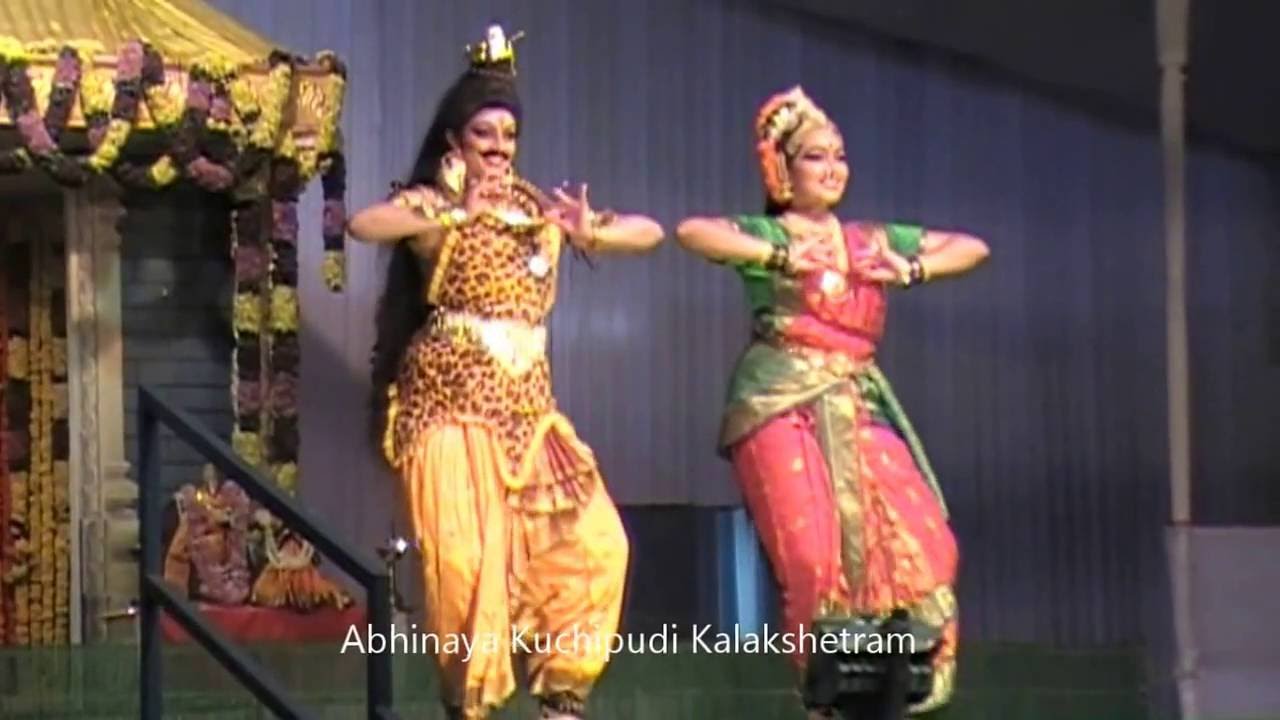This photograph, albeit of low quality and slightly blurry, captures an Indian ceremonial dance scene featuring two young women. Set against a backdrop of a large, gray-purple curtain and an ornately decorated gold gazebo structure adorned with floral garlands, the dancers perform on a wide stage or atop a staircase with a visible metal railing. Both women, appearing to be of Indian descent, are dressed in traditional Southeastern Asian attire, complete with intricate head wraps, ornate wristbands, bangles, and earrings. 

The dancer on the left wears a distinctive orange dress with a leopard print pattern on the upper portion and a crown-like headdress, complemented by her long hair. The dancer on the right is attired in a vibrant pink and green dress, accessorized with two bracelets on each hand. Their dance positions exhibit raised elbows at chest level, slightly bent knees, and a pronounced backward lean. The photograph includes a caption at the bottom, “Abhinaya Kuchipudi Kalakshatram,” presumably indicating the name of the performance or dance school, along with the photographer's name inscribed in white.